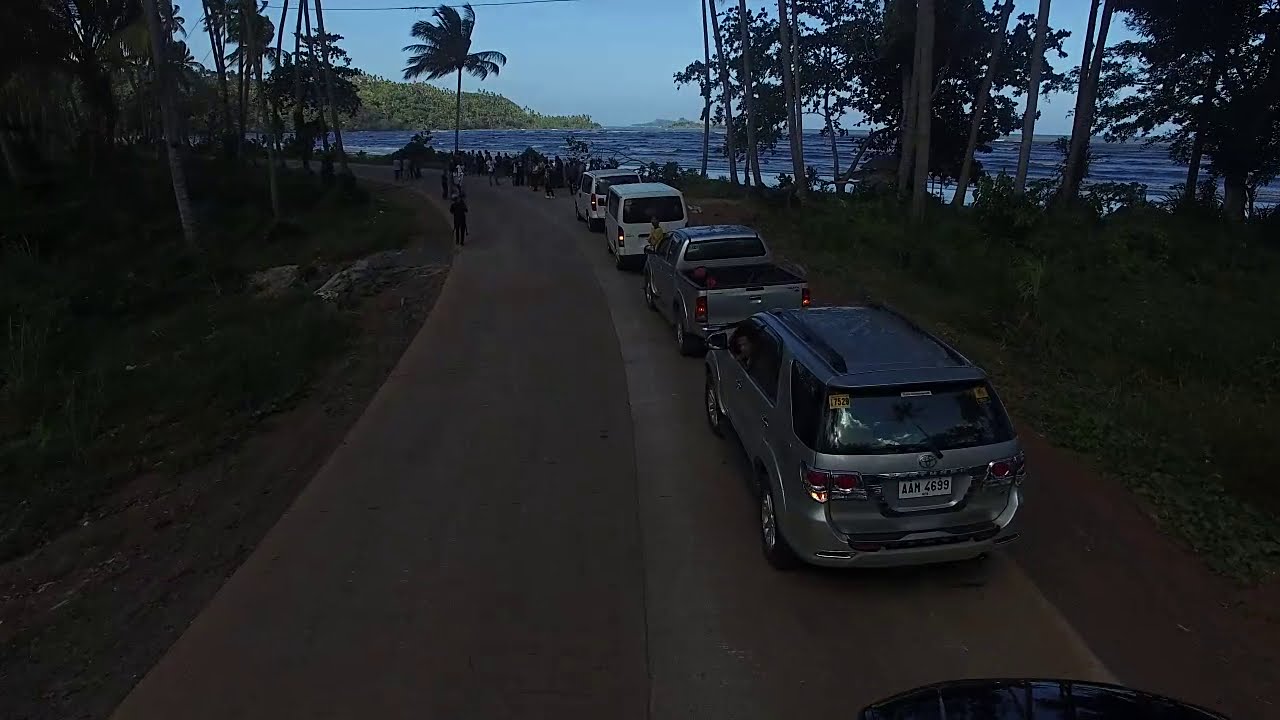The image captures a scene of five vehicles—including a gray SUV, a silver pickup truck, and two white vans—parked in a line on a paved road that curves leftward. The scene is set against a backdrop of a blue sky and appears to transition between bright daylight and the shadowed ambiguity of either an overcast sky or approaching dusk. This road, covered in patches of red dirt, is bordered by tall palm and pine trees, and lush green foliage on both sides. In the background, a cityscape and mountains are visible behind what seems to be an ocean or large body of water. A crowd of people is gathered in front of the vehicles near the trees, suggesting a social gathering near the tropical shoreline. The perspective from inside a fifth vehicle reveals part of its hood in the image’s foreground.